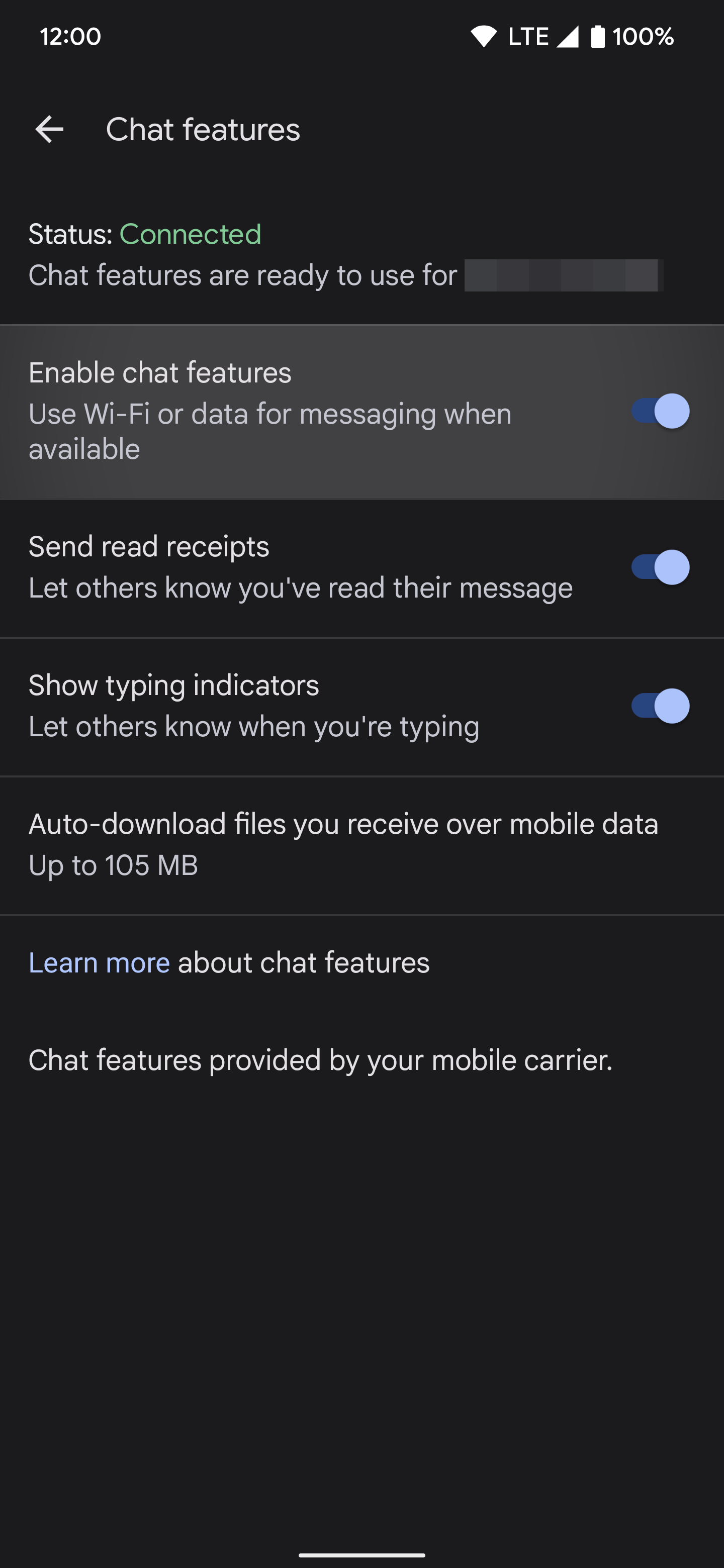This screenshot from a mobile phone displays a user interface in dark mode, with a charcoal black background. In the upper left corner, the time is shown in white font as "12." Over in the upper right corner, several icons in white font are visible: the Wi-Fi symbol, "LTE," the mobile signal strength icon, and a battery fully charged at 100%.

Just below, "Chat features" is labeled in white font, and to its left is a small white arrow pointing left. Directly under that, it states "Status: connected" in beige lettering.

In white font, the text below reads, "Chat features are ready to use for," but the subsequent information is censored with a gray paint overlay.

Further down, a gray rectangular section with white font indicates, "Enable chat features. Use Wi-Fi or data for messaging when available," which is toggled on. 

Below this setting, the screen presents options for messaging permissions:
1. "Send read receipts: Let others know you've read their message," toggled on.
2. "Show typing indicators: Let others know when you're typing," also toggled on.
3. "Auto download files you receive over mobile data up to 105 MB."

The display is organized with each functionality clearly defined and active.